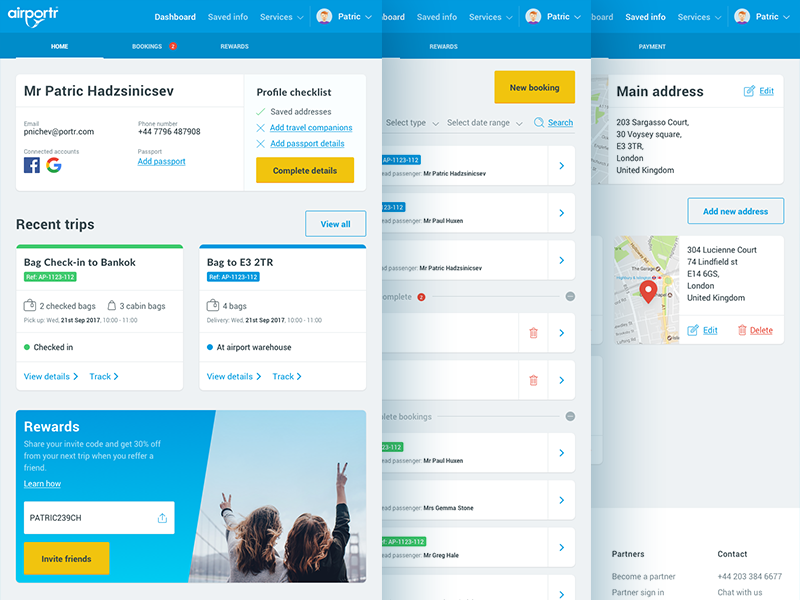The image displays a detailed view of a user interface for an application named "Airport R." The interface is designed to help users manage their travel-related activities. The screen showcases three pages, with the leftmost page being fully visible.

At the top of the interface, there are several navigational buttons labeled "Dashboard," "Saved Info," and "Services." To the right, there's an icon of a person with the partially visible text "Patrick," indicating the user is logged in.

The focus is on the "Home" tab, one of three main tabs which include "Home," "Bookings," and "Rewards." The home page displays the user's full name, Mr. Patrick Hadezanschweig, along with personal details such as his email and phone number. The section also shows connected accounts and offers an option to add a passport.

A profile checklist is prominently featured with tasks such as "Saved Addresses" (already checked), "Add Travel Companies," "Add Passport Details," and a "Complete Detail" button highlighted in yellow.

Further down, the page lists recent trips, with an option to "View All Recent Trips." It includes specific trip details like a checked bag to Bangkok at gate E32R, another bag with two checked bags, three cabin bags, and four total bags for another trip. The status of one bag is noted as checked in, while the other is marked as being at the airport warehouse.

At the bottom, there's a rewards section urging users to "Share your invite code and get 30% off your next trip when you refer a friend." Patrick's referral code, "Patrick23," is provided along with a call to action to refer friends.

The other images appear to show additional features and options for new bookings, but these sections are only partially visible.